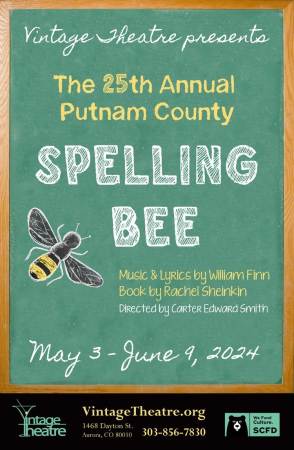This detailed poster depicts an advertisement in the style of a chalkboard, framed with wood as you would commonly see in a school setting. At the top, the cursive white text reads "Vintage Theater Presents," followed by "the 25th Annual Putnam County" in yellow serif font. The largest text on the poster boldly announces "Spelling Bee" in large white chalk-like letters. Just below this, there's a drawing of a bee, sketched to resemble chalk with yellow and black stripes and black wings. 

Continuing down the poster, yellow text states "Music and Lyrics by William Finn" and "Book by Rachel Sheinken," followed by "Directed by Carter Edward Smith" in white text. Below this, again in white cursive font, are the dates "May 3-June 9, 2024." 

The bottom section of the poster is black with blue labels and includes the website "VintageTheater.org," an address, and a phone number, providing all the necessary details for potential attendees. Overall, the poster mimics a chalkboard aesthetic with all its text and illustrations, making it a charming, illustrative promotional piece for the 25th Annual Putnam County Spelling Bee.